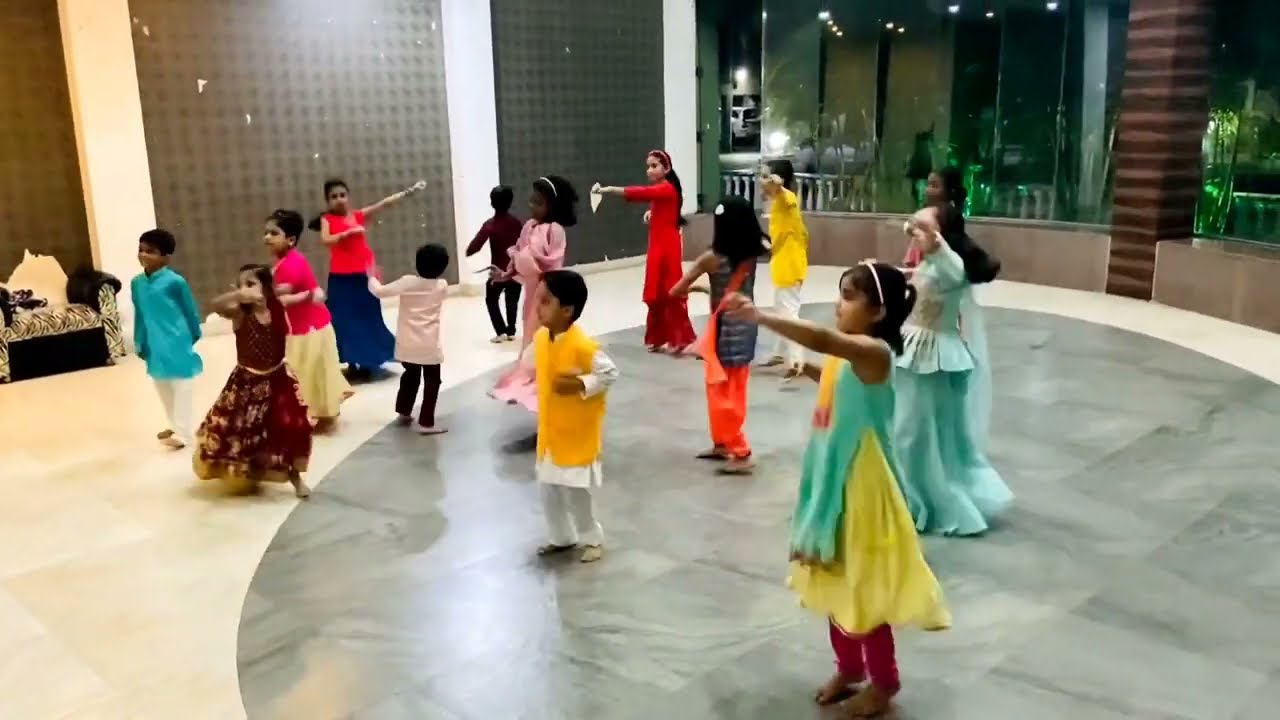The photograph captures a vibrant scene of about twelve young children, possibly ranging in age from 6 to 9, dancing in a large, circular room with a marble floor and a prominent gray circle in the center. The children, who appear to be of Indian or South Asian descent, are dressed in traditional clothing: the girls in long dresses of yellow, blue, red, and brown, and the boys in colorful two-piece outfits with long shirts and pants in hues of blue, orange, and gray. They all have their arms raised and knees bent as they move in unison, looking towards one direction. The room's design adds to the lively atmosphere, with brown and tan checkered walls on the sides, a glass wall at the back revealing a view outside, and a brown pillar along with plants visible in the background. The lighting reflects off the windows, illuminating the children as they perform. The image quality suggests it might be a screenshot from a video, giving it a slightly grainy appearance.